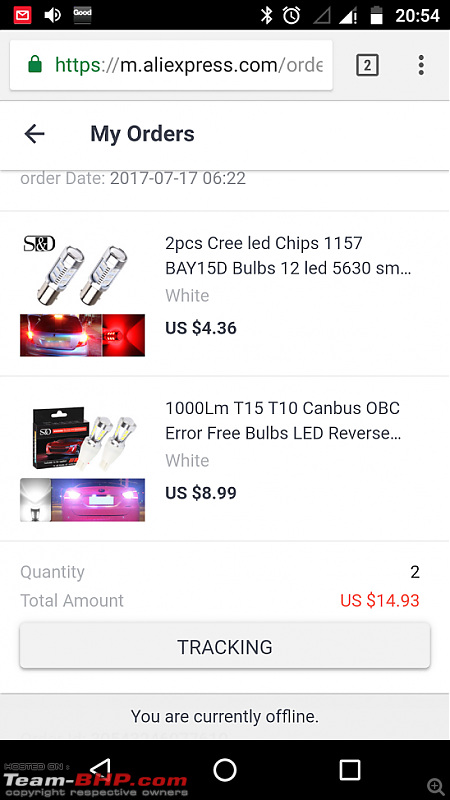Screenshot of a mobile AliExpress website displaying the order details page. The upper header includes standard mobile icons: an envelope icon on the far left, a red notification icon, a sound icon, and a 'Good' notification with a capital G in small letters. Moving right, there are icons for Bluetooth, alarm, a blank signal, a signal icon with an exclamation mark, a white square, and the time, which reads 20:54. 

Below the header is a search bar containing a lock icon, indicating HTTPS security in green, followed by the URL "https://m.aliexpress.com/order". To the right of the search bar is a square icon with the number two inside and a menu icon. Below that is a backspace icon and black text reading "My Orders".

A thin gray line separates these elements from the main content. The next section features the order date in uppercase letters: "DATE: 201707-170622". Below is a list of two ordered products, each accompanied by a tracking button. The total payment amount is shown in red as "US $14.93". A notification at the bottom states "You are currently offline".